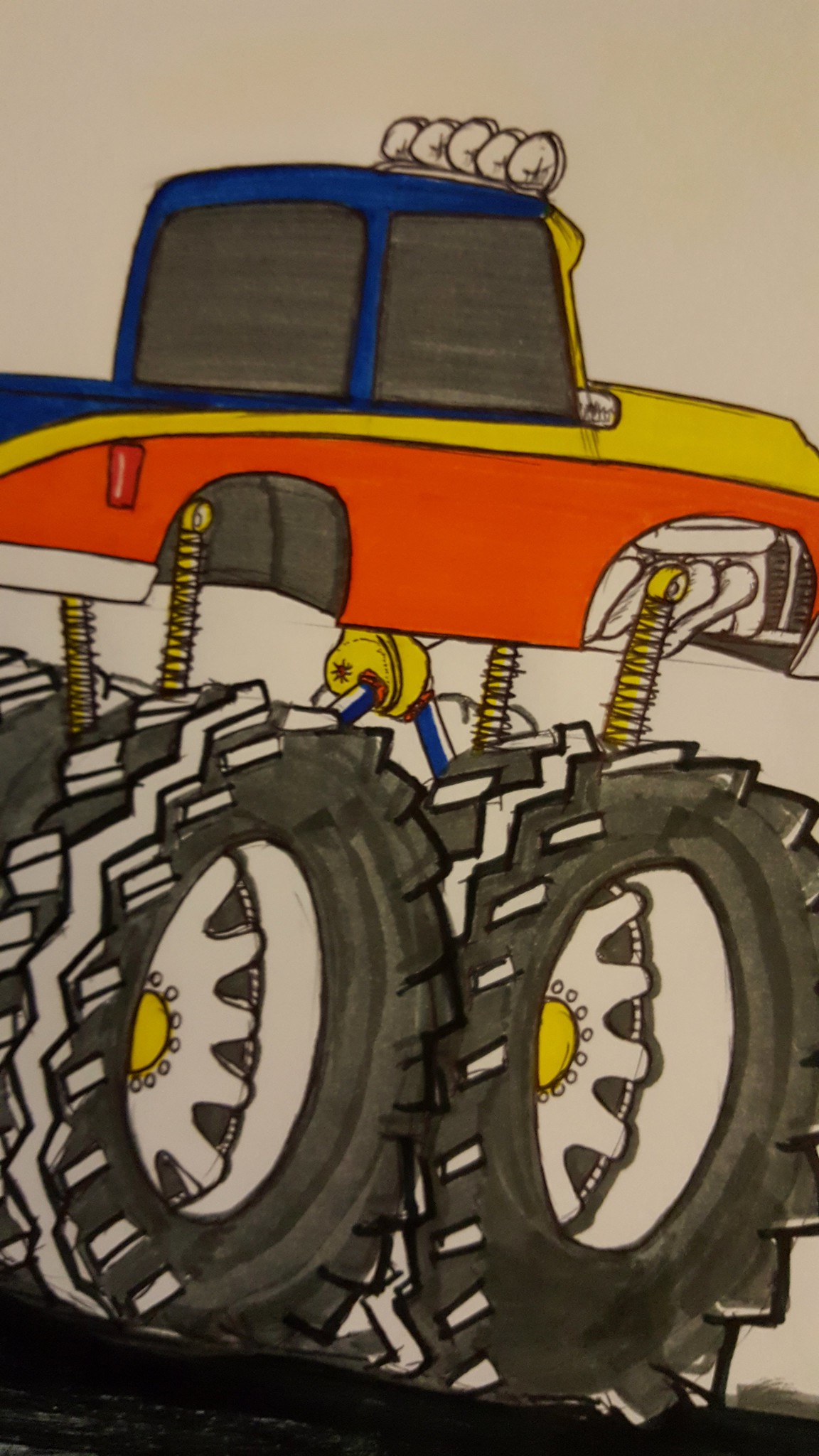A detailed sketch painting of a rugged, off-road truck in vibrant blue, yellow, and orange hues. The truck features five large, illuminated headlights mounted on its roof. It is equipped with massive tires, each connected via a visible hydraulic system that lifts the vehicle significantly off the ground. Attached to these tires are yellow tubes, adding to the mechanical complexity of the truck. Notably, the tires appear to be detached from the main body of the truck, highlighting the intricate suspension system. The tires themselves are black and white, with a distinctive yellow bolt pattern on the rims. The ground beneath the truck is depicted in striking black strokes, grounding the dynamic scene.